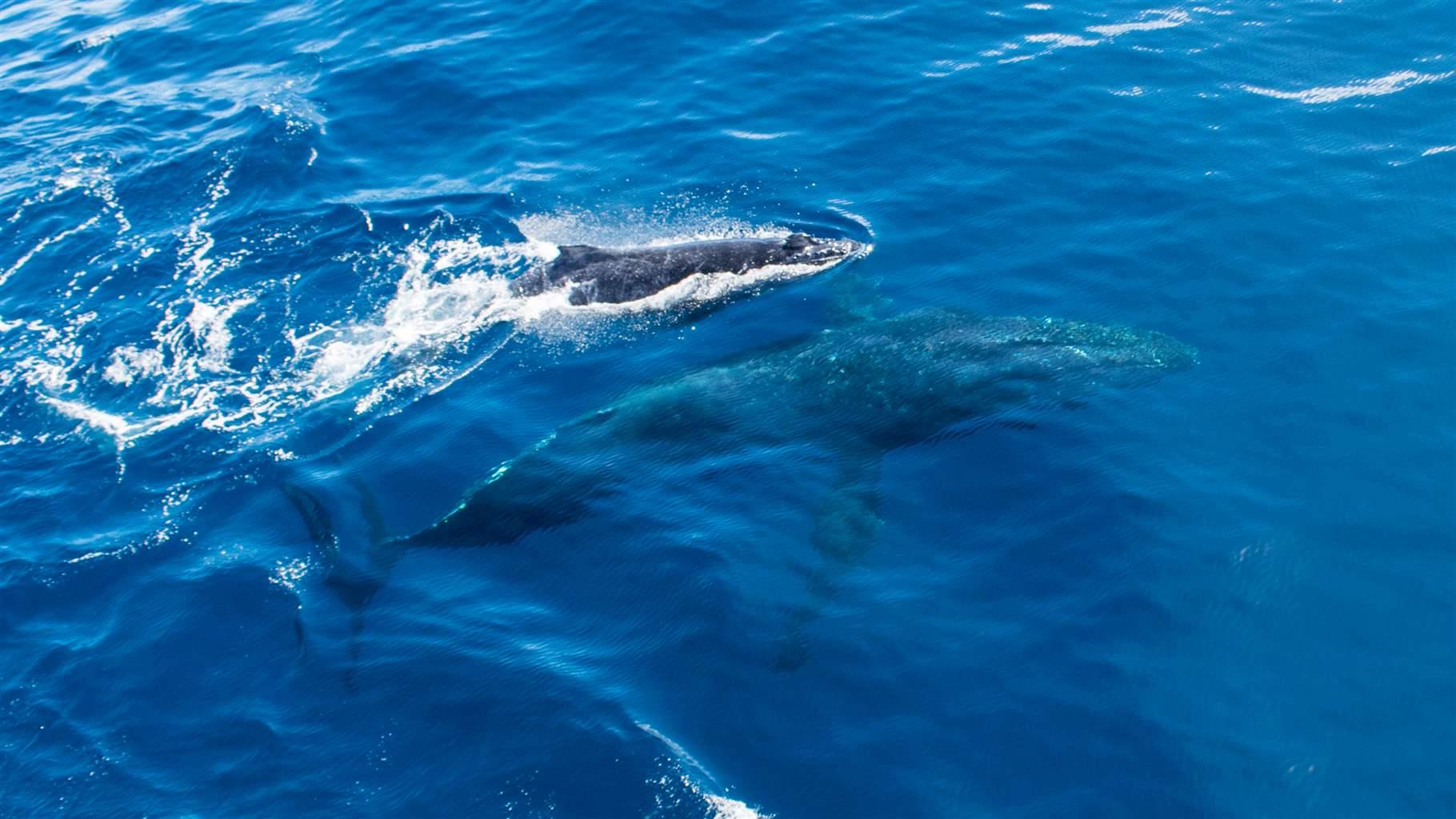This photograph, taken outdoors during the daytime from an aerial perspective, possibly by a drone or a large boat, vividly captures the serene blue ocean, which dominates the entire image. The water exhibits a beautiful medium blue hue with some darker blue tones at the bottom left. The photo is wider than it is tall, accentuating the expanse of the sea. In the top portion, a smaller sea creature—a dolphin or a young whale—has breached the surface, creating a series of white splashes and bubble waves. Adjacent to it, slightly submerged, is a larger sea creature, likely a whale, identifiable by its distinctive outline and wide tail, though its precise details are blurred by the water. Together, these creatures suggest a possible mother-and-baby duo gracefully navigating the ocean depths.